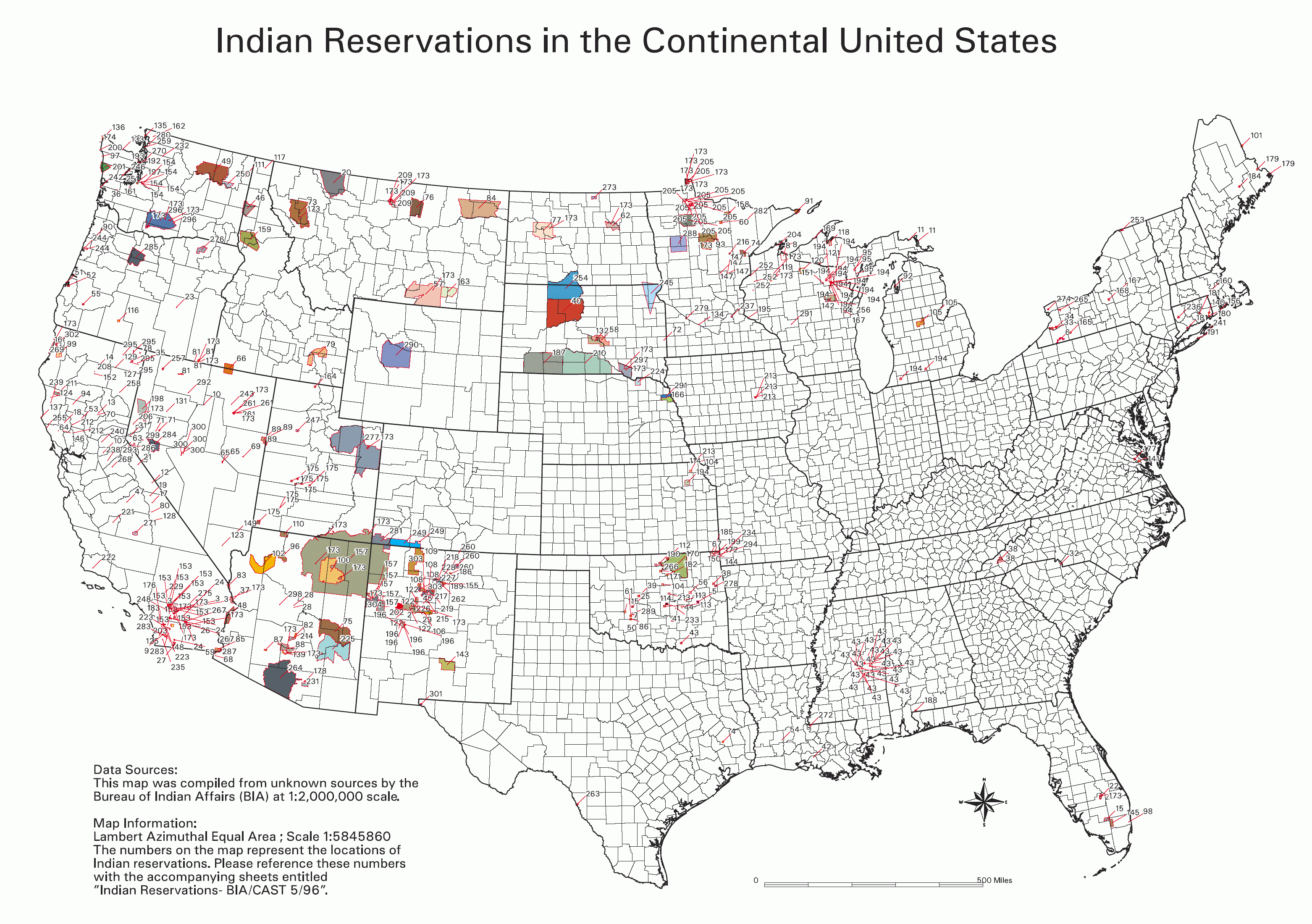The image is a comprehensive map of the entire United States, titled "Indian Reservations in the Continental United States" prominently displayed at the top. The map features various colored areas, predominantly situated in the western regions of the U.S., representing different Indian reservations. At the bottom of the map, there is a small, somewhat blurry paragraph that appears to mention a data source, likely the Bureau of Indian Affairs. Additionally, there is a note indicating "More Information," referencing certain numbers that were presumably provided for further details.